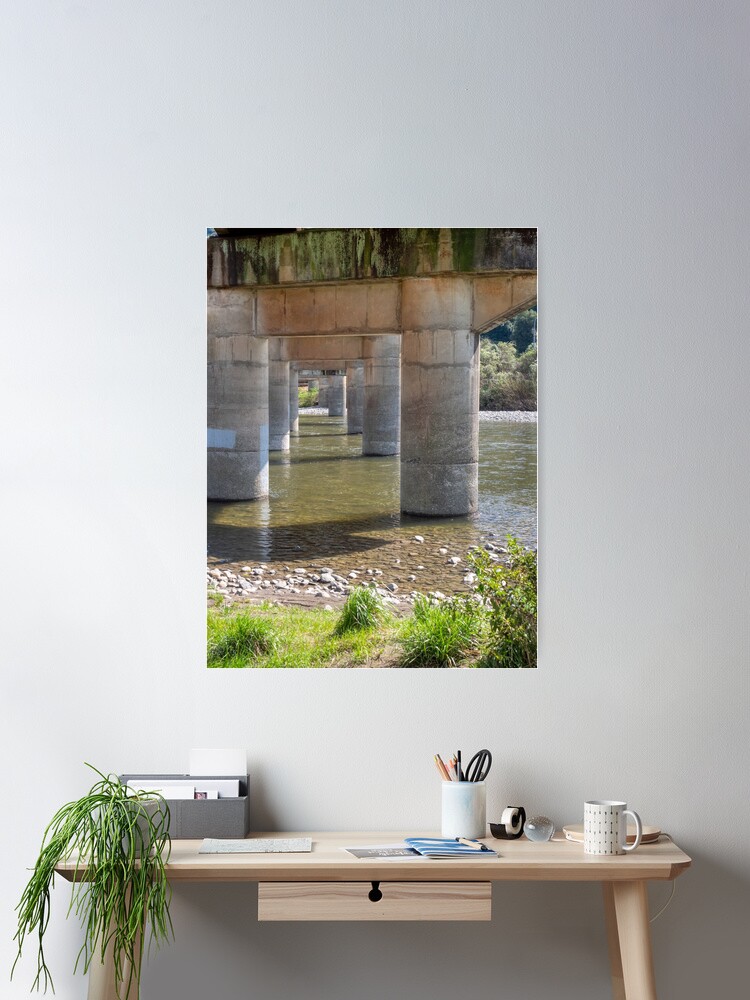The image features a light beige wooden desk with a single drawer in the middle, positioned against a large white wall. Atop the desk, a variety of office items are neatly arranged: a cactus plant drapes over the left side of the desk where a grey container with some folders is partially visible in the back. There is also a cup holding pencils and scissors, a roll of tape, a coffee mug, a few papers in the center, and a white lamp located towards the right of the desk. Mounted on the wall is a detailed photograph illustrating the underside of a bridge or pier. The image showcases cylindrical pillars rising from a shallow waterway, with green grass and rocks scattered around the base, stretching into the distance beneath the structure.